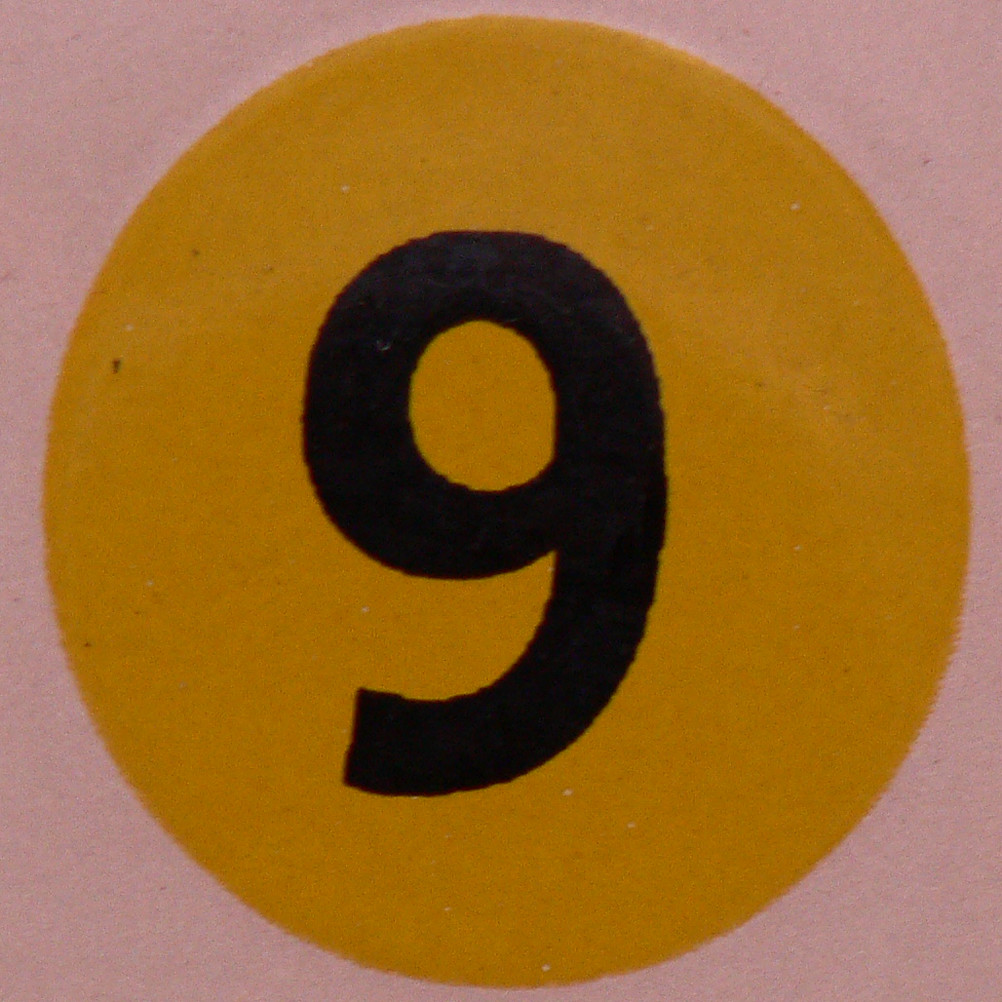In this image, we see a very large, solid yellow circle almost spanning the entirety of the frame, set against a light pink background. At the center of the yellow circle is a bold, black number that appears to be a 9, but its circular shape suggests it could also be a 6 if viewed upside down. The image quality is somewhat grainy, making it difficult to determine the medium, whether it's a photograph, a painting, or perhaps a close-up of an object like a button, sticker, or even candy. The number 9 has an old-fashioned, slightly cursive design, reminiscent of the style found on a bowling ball. The boundaries between the colors are not sharply defined, adding to the grainy texture of the overall image.